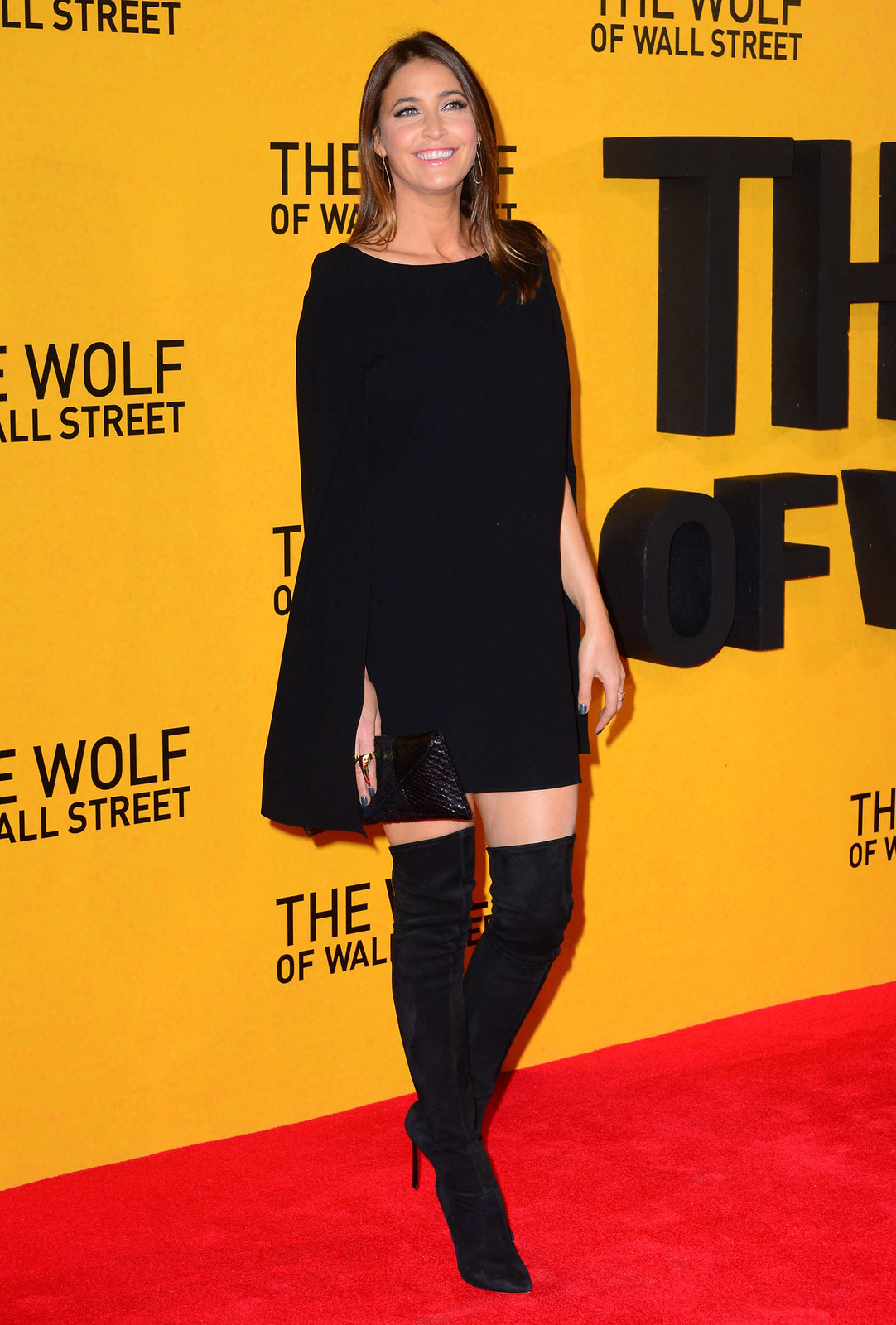In this detailed image, actress Lisa Snowden is seen arriving at the Wolf of Wall Street premiere held at the Odeon Cinema in London. She stands elegantly on a vibrant, bright red carpet, in front of a striking yellow backdrop adorned repeatedly with "The Wolf of Wall Street" text. Lisa looks stunning with her shoulder-length, honey-brown hair styled beautifully. She dons a chic black mini dress that features a dramatic cape-like back. Her ensemble is complemented by thigh-high, skin-tight, black stiletto boots, adding an edgy sophistication. She accessorizes with gold dangly earrings and multiple rings, accentuated by blue nail polish. In her right hand, she carries a textured, shiny black clutch. Lisa radiates confidence as she smiles off-camera, perfectly capturing the glitz and glamour of the red carpet event.